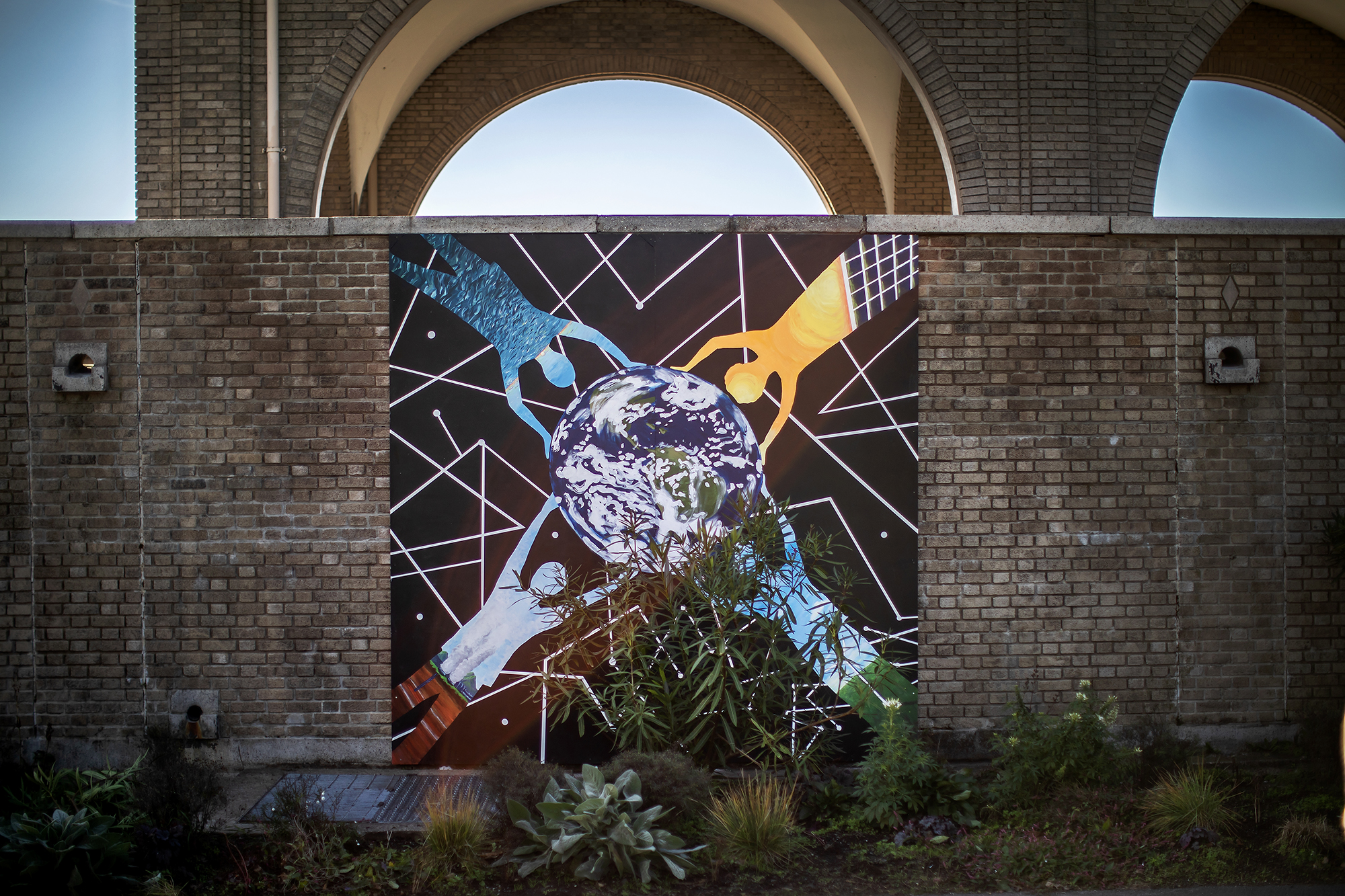The image depicts a vibrant and detailed mural painted on a low, brownish brick wall situated in an outdoor area, characterized by surrounding shrubs and ground grating. The mural itself is a large, square illustration featuring four human figures, each extending their arms towards the center to collectively support a painted Earth against a black background. Each figure occupies a corner of the mural, and is uniquely colored: the top left figure is blue, possibly representing the ocean; the top right figure is yellow, reminiscent of the sun; the bottom right figure is lighter blue with greenish pants, suggesting elements of water and land; and the bottom left figure is a bluish white with red pants, standing near a plant that partially obscures it. The mural is filled with small white lines that create geometric patterns and random dots that resemble stars. Behind this wall, there is a larger brick structure with archways, possibly part of a bridge or overpass, adding depth and context to the scene.